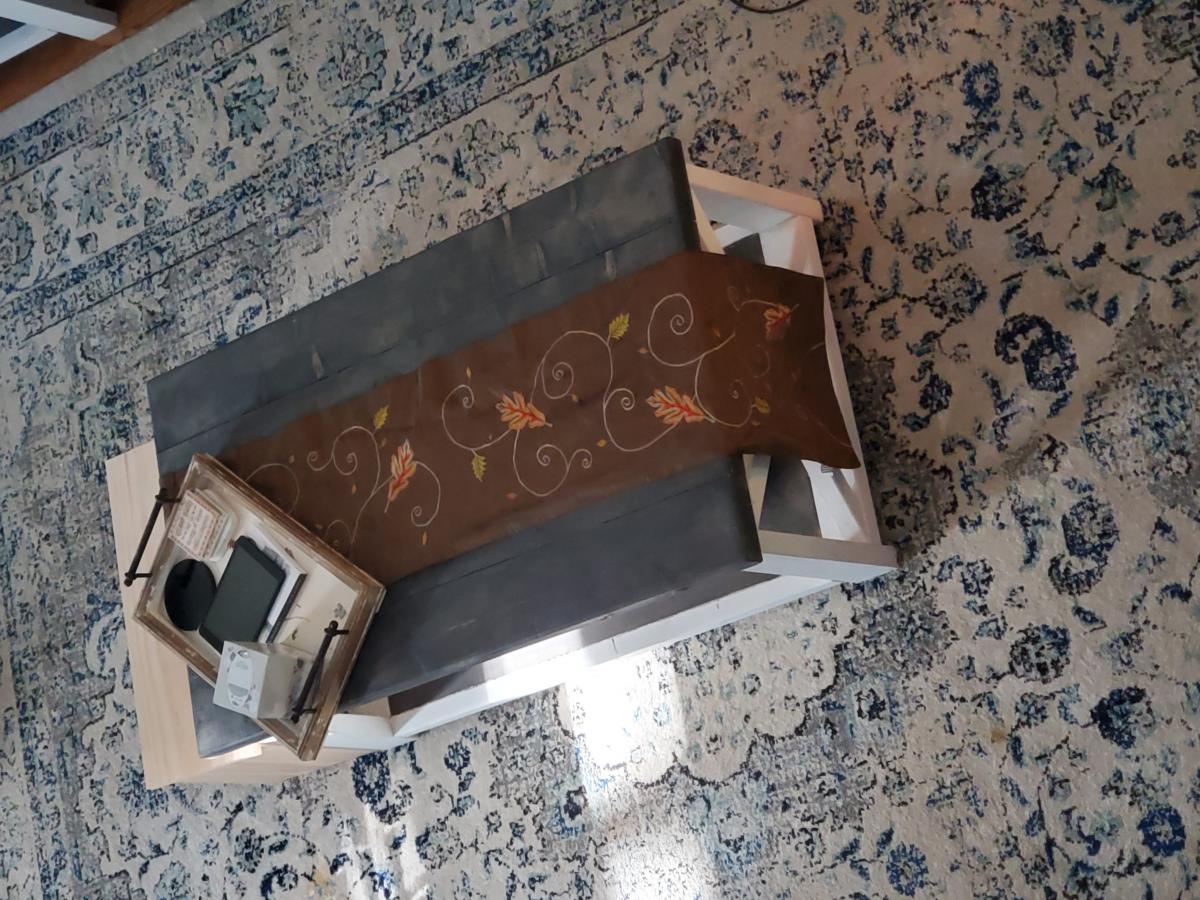In this photograph, a white and floral rug with a blue floral design pattern serves as the backdrop for the centerpiece of the room. The rug has a white base with intricate blue floral motifs scattered throughout. Placed centrally on the rug is a rectangular table. The table features a distinctive two-tone design: its base and legs are pure white while the tabletop is made from dark black wooden planks, creating a striking contrast. The tabletop is arranged somewhat diagonally, extending from the left to the right side of the photo towards the top right corner.

Adorning the center of the table is a decorative runner or blanket. This runner is rectangular, brown in color, and embellished with white floral spirals interspersed with orange leaves, adding a touch of elegance and warmth to the setting. Additionally, a small wooden tray with light brown finish and black metal handles rests on the table. This tray holds a few items: a large electronic tablet, reminiscent of an iPad, and a white tissue box. The overall arrangement provides a harmonious blend of colors and textures, accentuating the room's cozy and stylish atmosphere.